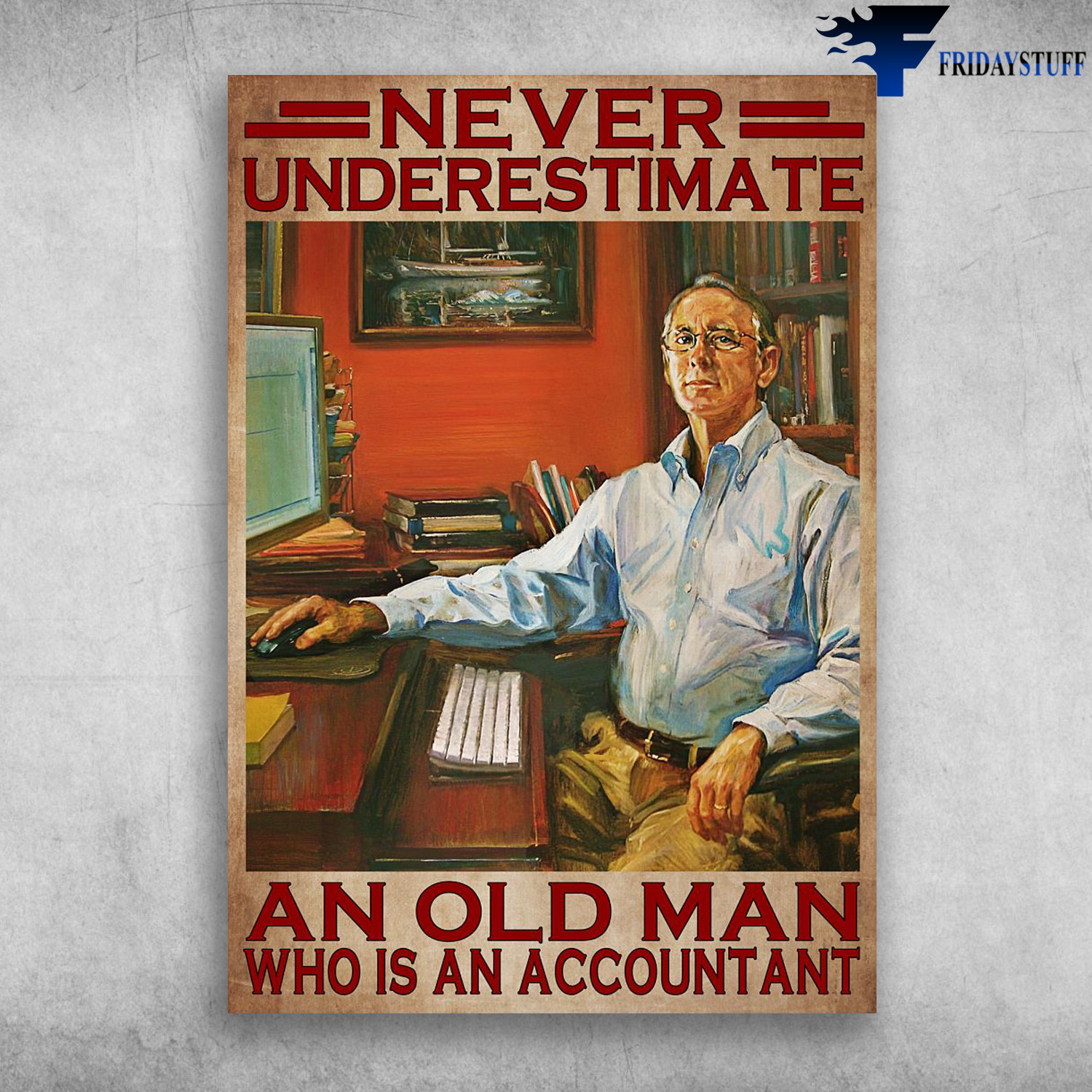This image features a detailed, photorealistic illustration of an elderly man at a computer. The focal point is a poster that prominently displays the phrase "Never underestimate an old man who is an accountant" at both the top and bottom sections. The man depicted in the illustration has a very stern, authoritative expression. He wears glasses, a light blue shirt, and beige/tan pants, and he is using a wireless mouse while working at his desk. The desk holds a white keyboard and the computer screen, and the background showcases his office environment complete with a personal library and a painting of a boat on a red wall. Additionally, in the upper right corner of the image, there’s a distinctive logo featuring the letter 'F' with flames emanating from it, accompanied by the text "Friday Stuff."